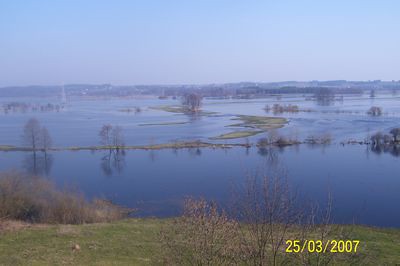The image captures a serene swamp landscape with a slightly hazy or blurry atmosphere. In the foreground, vibrant green grass and scattered shrubs are visible, giving way to a marshland predominantly covered in water. Sporadic trees and shrubs emerge from the water, some appearing on small sandbars with patches of higher land. The water, reflecting a blue hue, blends seamlessly with the rolling hills in the distant background, which are also a shade of blue, creating a cohesive and calming color palette. Above the horizon, the sky features a subtle mix of blue and white tones, enhancing the overall hazy appearance. The entire scene suggests it was photographed from a higher vantage point, possibly a grassy hill overlooking the marsh. In the bottom right-hand corner, a date stamp in yellow reads "25/03/2007," indicating when the picture was taken. The composition harmoniously balances elements of water, greenery, and sky, making it a captivating yet tranquil snapshot of nature.